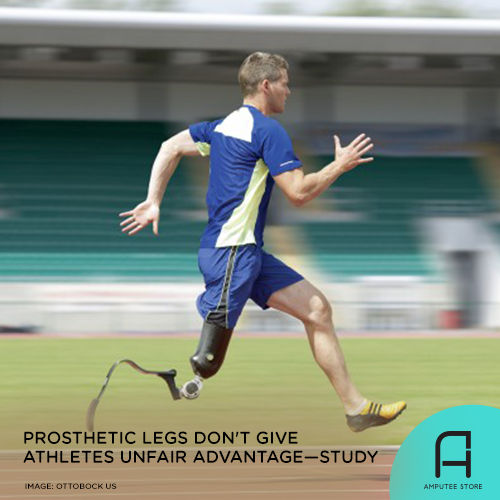This color photograph captures a paraplegic man running swiftly towards the right. He wears a distinctive blue shirt adorned with yellow accents at the armpits and white detailing on the top back and front. His outfit is completed with blue shorts featuring a black stripe that runs down to his black prosthetic leg. His right leg is a blade-type prosthetic, characterized by its black attachment at the thigh and a metal arc shape, while his left leg is clad in an ankle-length yellow sneaker with black accents and three black stripes. The man’s arms are dynamically positioned, with his right arm bent forward and his left arm bent back, indicating vigorous motion. The background of blurred stadium seating enhances the sense of speed and movement. Superimposed at the bottom left of the image is text reading, "Prosthetic legs don’t give athletes an unfair advantage – study." Below this, it says, "Image: Ottobock US." Additionally, in the bottom right corner, a small cyan semicircle encloses a stylized 'A' with the words "amputee store" written beneath it.